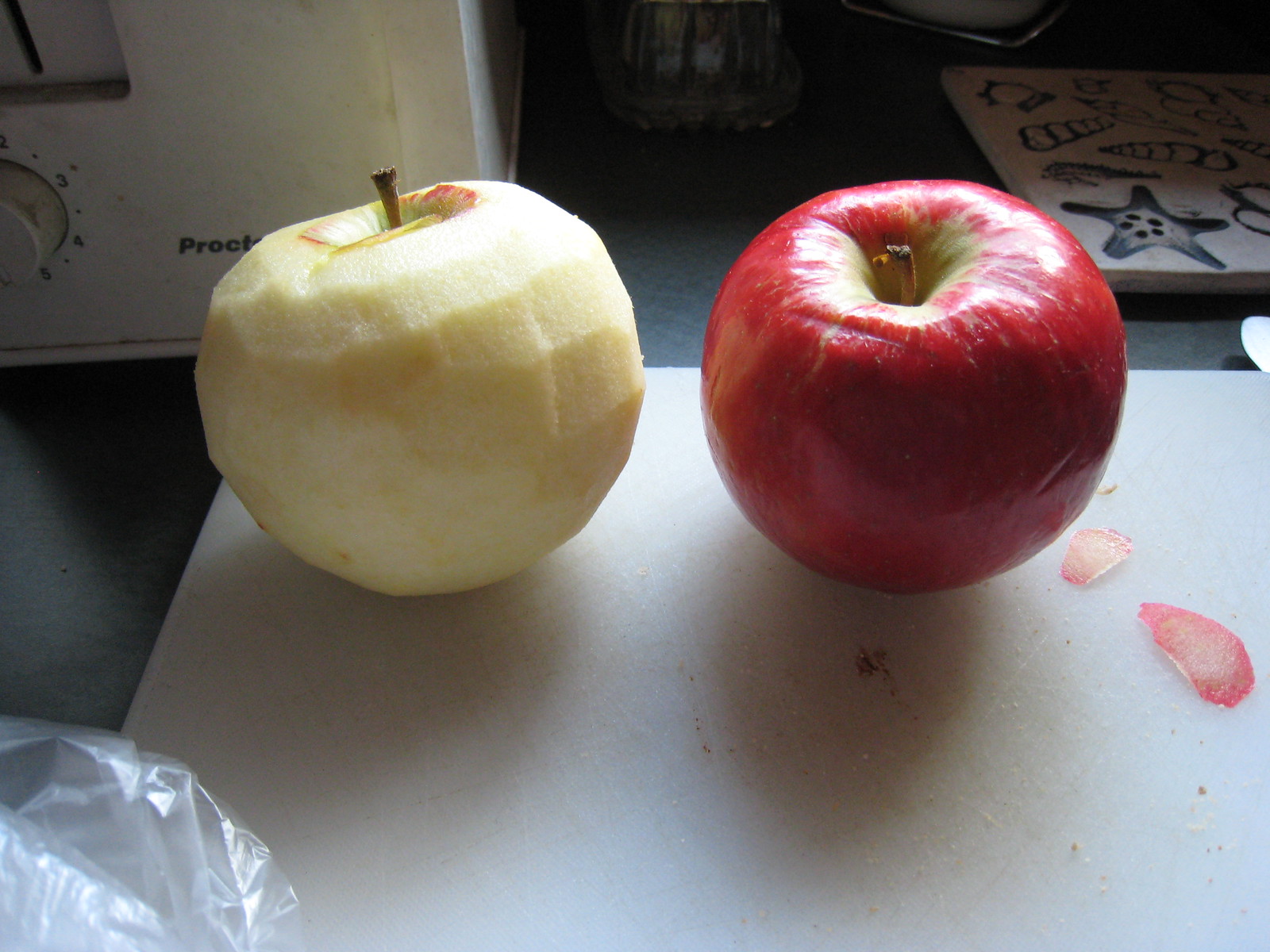An indoor, close-up color photograph captures a scene on a gray countertop. At a downward angle, the image prominently features a plastic cutting board centered amidst various kitchen items. To the left of the cutting board is a completely peeled apple, its whitish flesh fully exposed, while to the right, a fresh red apple remains unpeeled. Both apples have their stems pointing upwards, indicating their freshness. Scattered bits of apple peel lie just below the unpeeled apple, extending towards the right edge of the frame.

In the background to the left, part of a white toaster is visible, with its control knob showing the numbers three, four, and six around the dial. On the right side, a square potholder adorned with seashell patterns can be seen. Near the lower left edge of the image, part of a reflective plastic bag is visible, catching some light from the nearby source.

The primary light source originates from the upper right, illuminating the tops of both apples and casting shadows to the left. The area in the center-right background is devoid of distinct details, shrouded in darkness, save for the visible kitchen elements. The photograph captures a simple yet vivid moment in a kitchen, focusing on the contrast between the peeled and unpeeled apples.